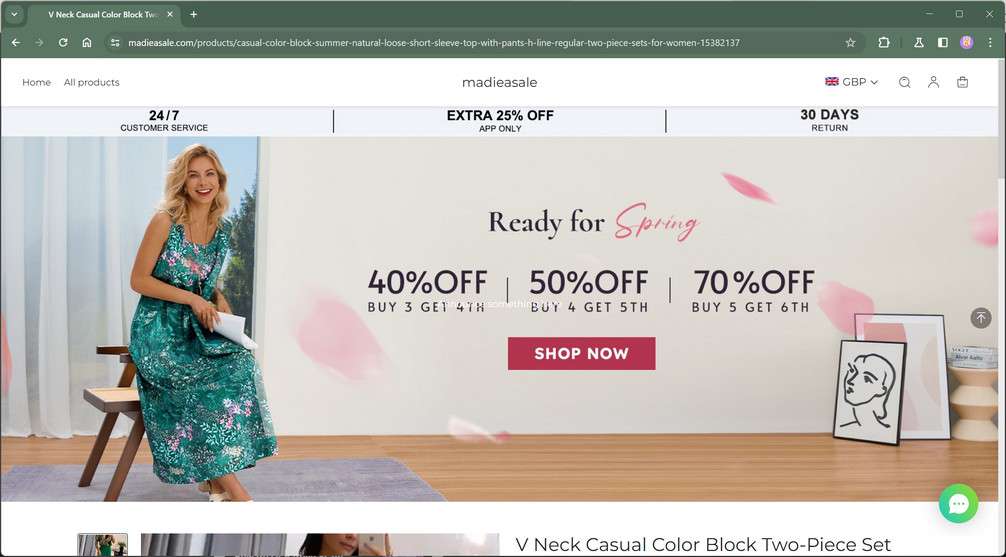Image Description: 

The image is a screenshot of a clothing store’s website, Maddy's Sale. At the upper left corner of the screen, there is a browser tab labeled "V-Neck Casual Color Block". The browser’s navigation bar, which includes the back, forward, refresh, and home buttons, is visible beneath the tab.

The web address displayed is "maddyasale.com/products/casual-color-block-summer-natural-loose-short-sleeve-top-with-pants-h-line-regular-two-pieces-two-piece-set-for-women".

Below the address bar, there is a menu, followed by the main window showcasing the webpage's content. The primary image in the main window features a woman sitting on a chair, facing the camera with her body angled slightly to the lower right. The text to the right of the woman reads "Ready for Spring" and highlights the promotional offers: "40% off, Buy Three, Get Fourth Free", "50% off", and "70% off".

The webpage appears well-organized and focuses on promoting the featured casual color block summer attire for women.